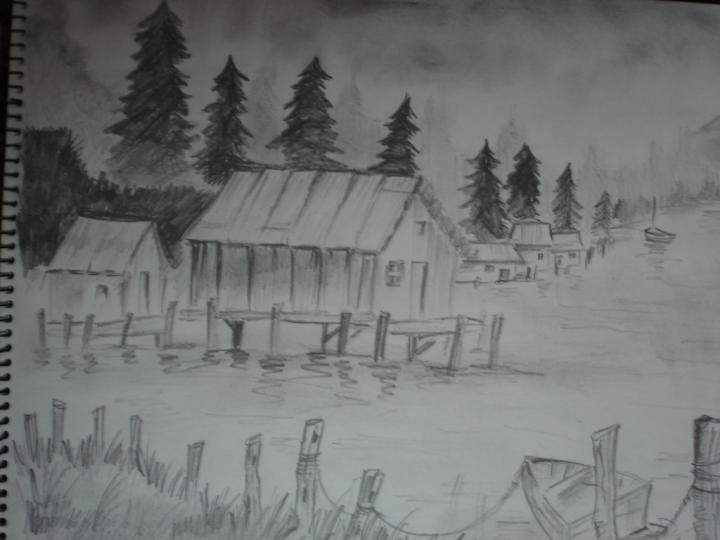This pencil sketch appears to be a detailed illustration from a "Learn to Draw" book, created on a sketch pad with binding on the right side. The scene depicts a serene lakeside setting featuring two rustic cabins and accompanying docks. In the background, the sky is shaded in a gradient of gray and white, lending a tranquil ambiance to the image. A collection of fir trees lines the horizon, varying in size from larger on the right to smaller towards the left, adding a sense of depth and perspective.

In the foreground, there is marshland accentuated by a small, brown fence. The water is illustrated with gentle ripples, suggesting a slightly disturbed surface. On the left-hand corner, a tiny, triangular boat is partially visible, while another boat floats further away on the lake. Scattered along the shoreline are additional sheds or cabins, increasing the complexity of the lakeside community scene.

Further enhancing the depth, some of the fir trees are smudged, creating a layered effect. This detailed composition captures the essence of a tranquil fishing lake, complete with various buildings, boats, and natural elements, all meticulously rendered in pencil.